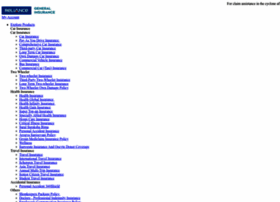This is a moderately blurry image with indistinguishable details upon zooming in. The top of the image has a gray border featuring black text on the top right and a dark blue button below and to the left. Next to the blue button, there are five clickable areas followed by three gray buttons on the right. Two of the gray buttons are significantly larger—approximately four times the size of the smaller one. Further to the right, there's a prominent orange button. The background is a light gray, and on the left side, there is a marketing slogan stating, “Live worry-free, live smart, get world-class protection with our automobile plans.”

Below this slogan, there are three lines of text, each accompanied by an icon. Additionally, there's an illustration depicting the world with visible continents and oceans, alongside a blue robot-like character walking across it. This robot has yellow arms and legs, and is wearing blue shoes. The bottom of the image features another line of text that reads, "Why Choose Reliant General Insurance." On the right side of the image, there's a box containing four clickable areas with a text box positioned beneath them.